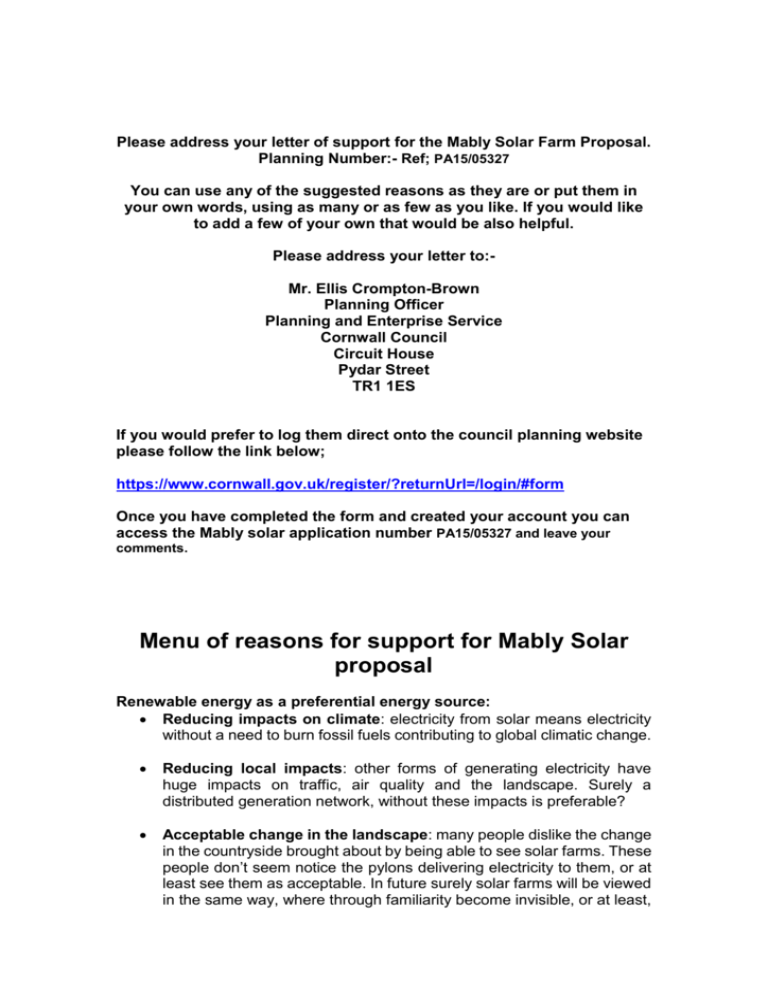This vertical image features text on a white background, with no border, and is divided into distinct sections. At the top left corner, the text begins with "Please address your letter of support for the Mabley Solar Farm proposal" followed by the planning number. It encourages the reader to use the suggested reasons for support verbatim or to rephrase them, and also suggests adding personal reasons if desired.

Beneath this, the text instructs the reader to address their letter to a specific recipient, shown in centered text. It then provides an alternative method for submitting comments directly on the council's planning website, followed by a blue hyperlink: "www.cornwall.gov.uk/register" with additional text indicating steps to create an account and access the Mabley Solar Farm application number to leave feedback.

In bold black text, a section labeled "Menu of Reasons for Support for Mabley Solar Proposal" follows. This section includes a heading: "Renewable Energy as a Preferential Energy Source," under which three bullet points are listed:
1. Reducing impacts on climate
2. Reducing local impacts
3. Acceptable change in the landscape

Each bullet point is accompanied by further explanatory text.